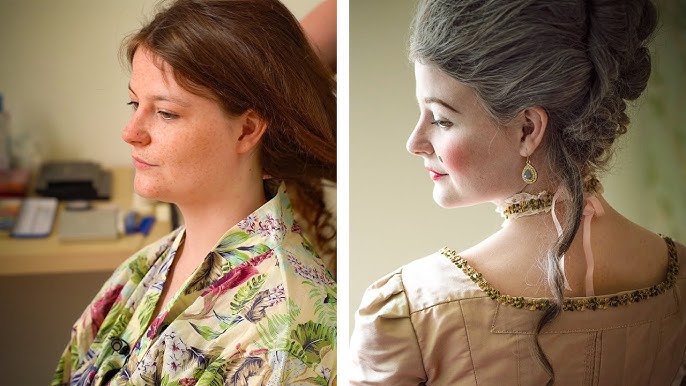The image is a side-by-side before and after self-portrait featuring the same woman. On the left, she has long, reddish-brown hair and is wearing a floral robe or blouse with green leaves and red and purple flowers. She is sitting with her body slightly turned to the side, facing left, and someone is working on her hair; part of their arm is visible. Her natural appearance includes no makeup and her hair is down. In the blurred background, a desk or table with indistinct items can be seen. In the right image, the woman is transformed, styled to emulate a character from a period piece. Her hair, now a grayish-black, is elaborately put up, and she wears heavy makeup with white face powder, rouge, red lipstick, and a painted beauty mark. She sports drop earrings and a tan Victorian gown with a greenish-gold border around the collar, paired with a matching choker tied with a pink ribbon. The photo captures her profile, facing sideways, with the sun shining on her face, illustrating a dramatic before and after.